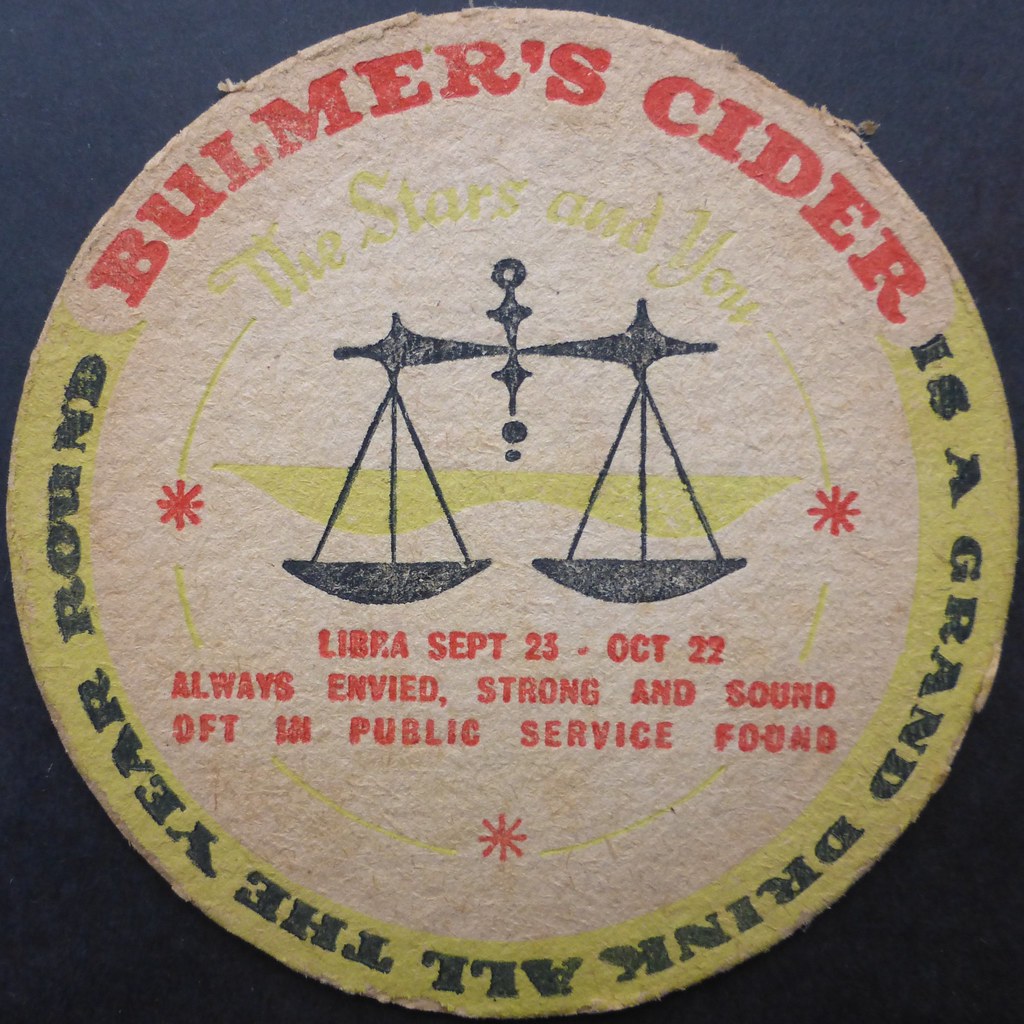The image showcases a circular, worn-looking coaster set against a dark blue background. The coaster features intricate designs and a wealth of text detailing both a promotional message and astrological content. At the top, in bold red lettering, it reads "Bulmer's Cider." Circling around the edge from the top right is a black inscription stating, "is a grand drink all the year round," set against a yellow perimeter that encompasses roughly two-thirds of the coaster's bottom. Just below the top, in yellow text, the words "The stars and you" are framed by two lines extending downwards, each ending in a red star symbol. Dominating the center of the coaster is an image of a traditional weighing scale, evenly balanced and depicted in black with a yellow backdrop. Directly beneath the scales, more red text proclaims "Libra September 23 through October 22," followed by the phrase "always envied strong and sound, oft in public service found." Further enhancing the design, additional red asterisks are positioned around the central image and near the bottom edge of the coaster.